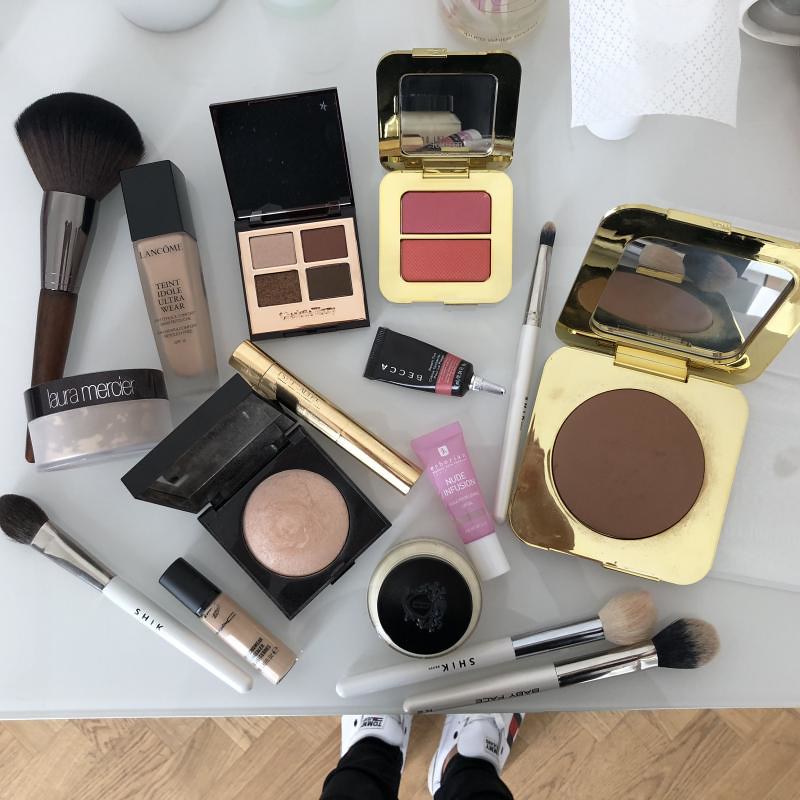A brown wooden floor provides the backdrop for the scene, where a person is partially visible, standing with their feet clad in white shoes and legs in black pants. They are positioned under a white table. The tabletop is cluttered with various makeup products, including several blush sticks and a mix of makeup palettes. Among the palettes, some are specifically for eyeshadow while others contain blush, showcasing different shades of brown, pink, and red. Notably, there is a tube labeled "foundation" and an eyeshadow stick present. The blush colors range from beige to brown, and the eyeshadow palettes feature an array of hues, enhancing the variety of cosmetics on display.